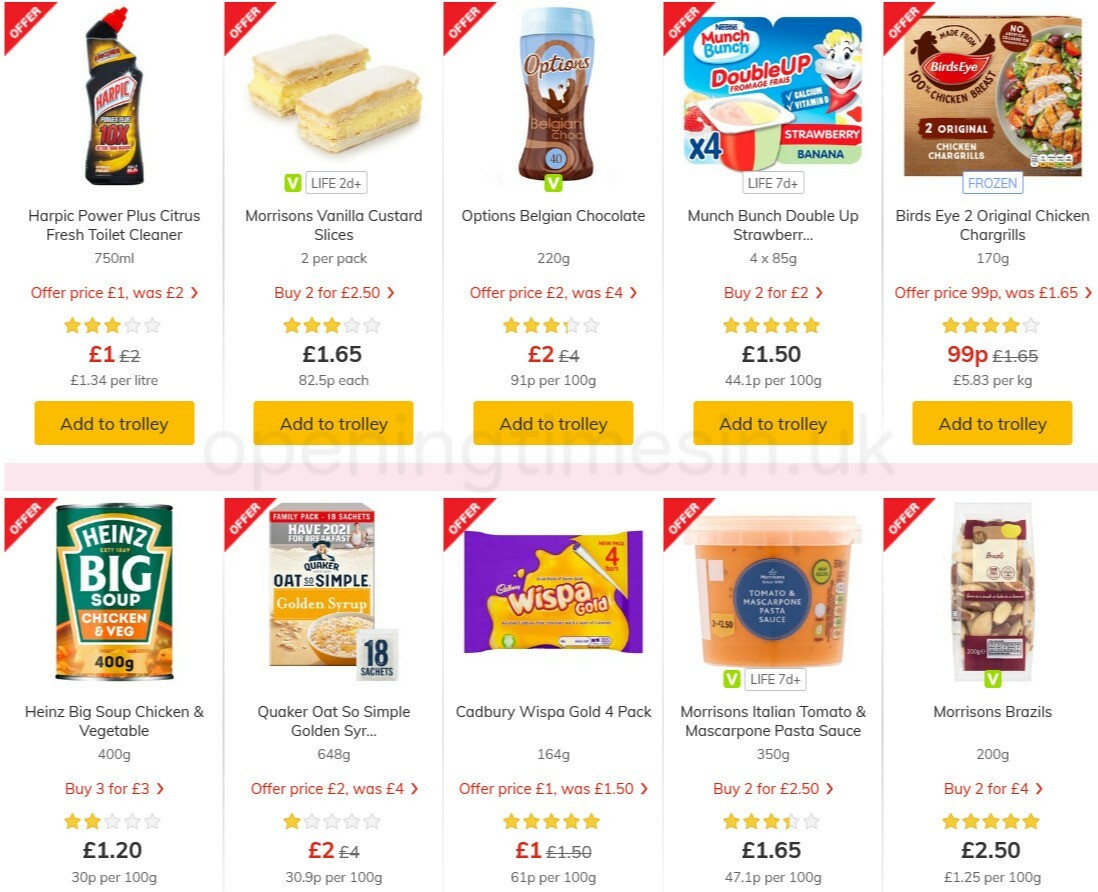This image showcases a vibrant online grocery shopping interface featuring a selection of ten food items. The website layout is designed to allow users to easily add items to their cart and proceed to checkout. 

In the first row, there are five distinct products:
1. **Fresh Toilet Cleaner** - This item is showcased with a clear image and a comprehensive description, including its volume in liters or milliliters. 
2. **Vanilla Extract** - Presented with detailed measurements and specifications.
3. **Vanilla Custard Slices** - A delicious treat displayed with its size and serving information.
4. **Belgian Chocolate** - Highlighted with its weight and quality details.
5. **Munch and Bunch Double Up Strawberry Yogurt** - Featuring nutritional information and quantity.

Each product in the first row has an area that specifies:
- The original price and any current offer price.
- A rating, depicted with stars, showcasing customer reviews.
- The price per unit or per liter.

At the bottom of each item's description, a yellow rectangle button labeled "Add to Trolley" makes it easy for shoppers to add products to their cart. 

The second row also features five items, although the bottom part of this section, including the "Add to Trolley" button, is cut off:
1. **Heinz Chicken and Vegetable Soup** - Displayed with its volume and nutritional content.
2. **Quaker Oats** - Detailed with serving size and health benefits.
3. **Cadbury Gold Four-Pack** - Highlighting its quantity and price per pack.
4. **Pasta Sauce** - Presented with its weight and flavor description.
5. **Brazil Nuts** - Showcased with information on weight and nutritional benefits.

Each item on the website includes a picture, detailed description, price, offer information, and a rating system. The prices are listed in pounds, and the cost is broken down per liter or per unit, ensuring shoppers have all the information needed to make an informed purchasing decision.